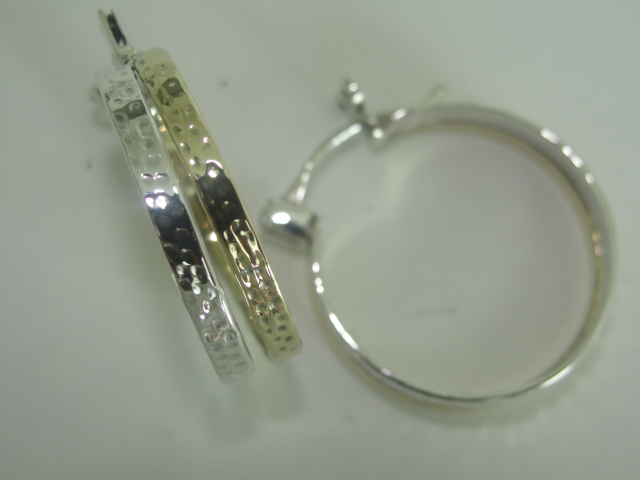The photograph captures a set of three intricate jewelry pieces, likely earrings, displayed on a white background. On the left, there are two ring-like items, each featuring a distinct dot-like pattern imprinted on their surfaces. The first ring on the far left is made of silver and exhibits a slightly stamped appearance with small circular indents along its reflective surface. Adjacent to it is a golden ring, possibly bronze or rose gold, sharing a similar imprinted circle design. On the right side of the image lies a third jewelry item, another shiny silver ring, distinguishable by its clasp mechanism, clearly indicating its use as an earring. This third piece also has an attachment with a small thin pole, catching the light at the top, while the background highlights its sleek, polished finish. The interplay of light reflecting off these metallic surfaces adds a layer of sophistication and detail to the overall presentation.